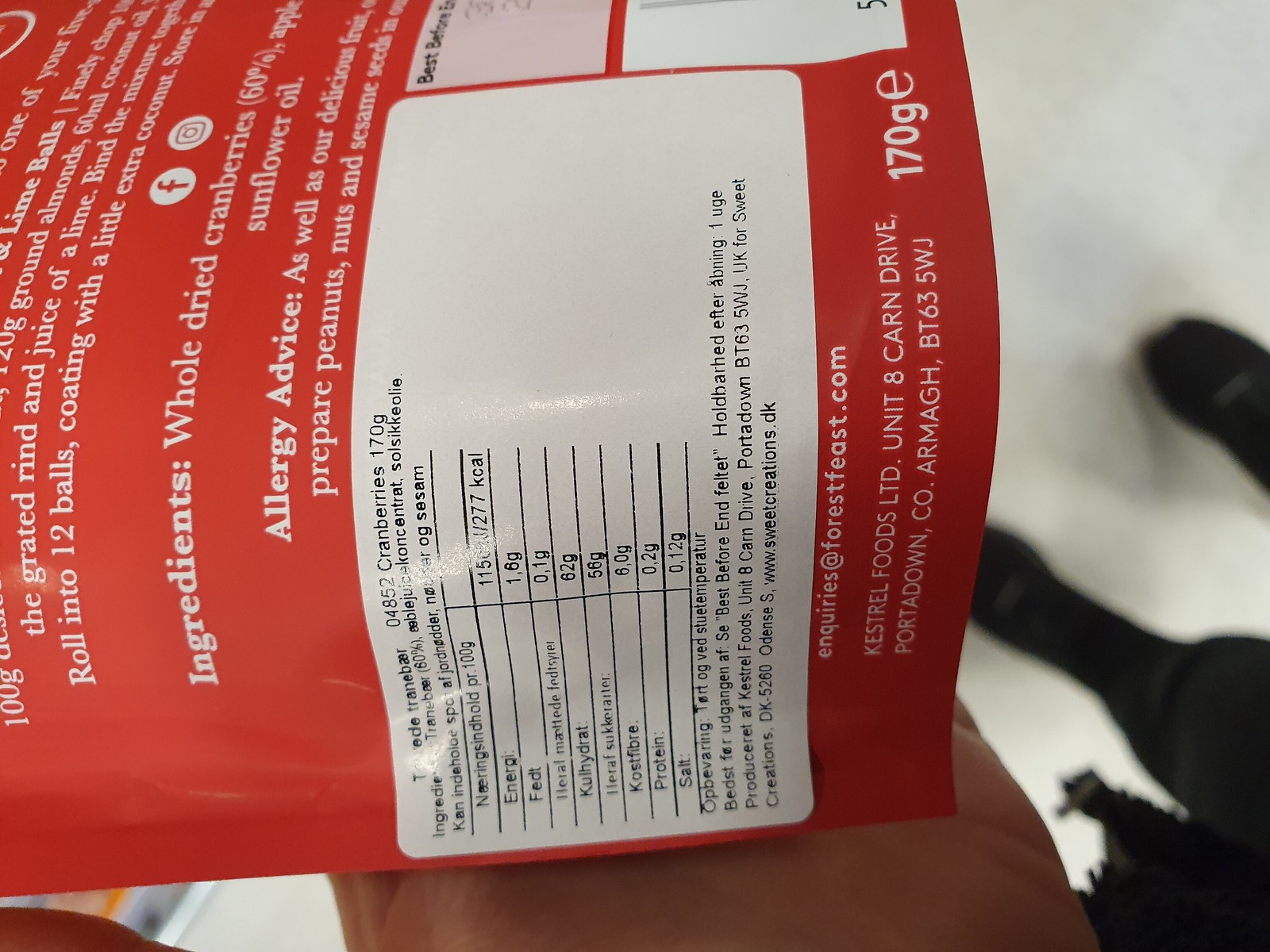This is a detailed photograph taken indoors, showing the back of a red packet of whole dried cranberries, held by a person from above. The packet features a prominent white rectangular sticker in the middle, displaying nutritional information primarily in white text, with some words highlighted in red. Additional text on the packet includes a list of ingredients (notably including sunflower oil), allergy advice warning of possible nut contamination, and an address indicating it's made by Kestrel Foods Limited on Kern Drive in Portadown. The packet also displays a weight of 170 grams and features logos for Facebook and Instagram. The image is oriented 90 degrees counter-clockwise, and you can see the person's legs on the side.